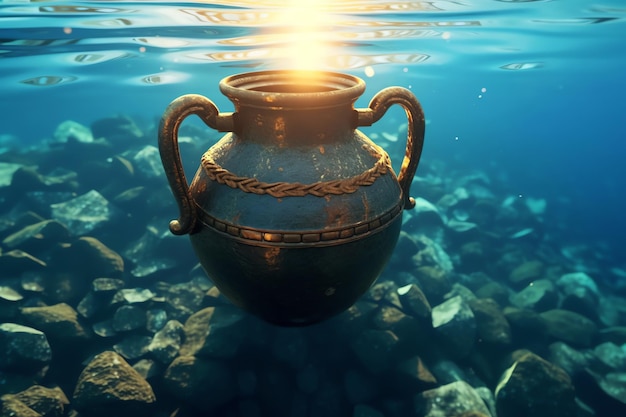The image captures a scene underwater with a striking urn as the focal point. This urn, or pot, is distinctly round with two elegant, arching handles on either side. It boasts a blue or blue-green hue adorned with faded golden details, showing its age through patches that resemble rust and scratched-off paint, revealing darker tones underneath. A bright yellow beam of light illuminates the urn's top, emphasizing its intricate design. This scene is set against a backdrop of clear blue to dark blue water, with numerous rocks beneath the urn. The top of the image features a wave pattern, precisely positioned just above the urn without obscuring it, allowing for a clear view of both the calm surface and the underwater details. The water’s surface reflects light and ripples, adding to the surreal quality of the photograph, which appears digitally retouched to highlight these juxtaposed elements. Despite the clear water revealing every stone and ripple, no fish are present.